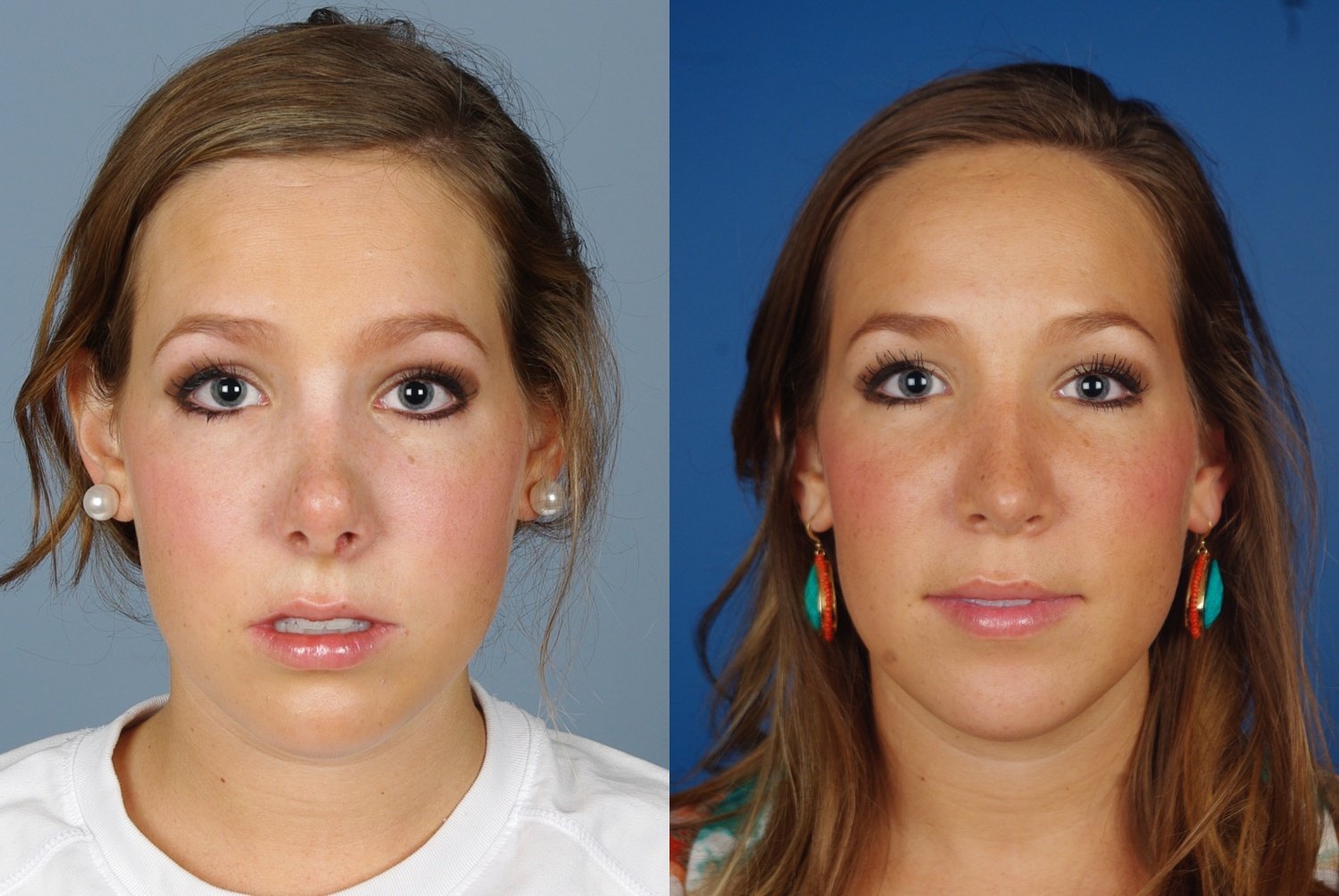This image is a before-and-after comparison of a young woman, showcasing a significant transformation. On the left side, she appears in front of a light blue background, wearing a white t-shirt and small pearl earrings. Her hair is pulled back into a ponytail or bun, with a few wisps falling around her face, and her expression looks scared or anxious. Her makeup is minimal, though she does have mascara and eyeliner, giving her eyelashes a longer appearance. Her face is pale, and the photo is a close-up, focusing on her neck upwards.

The right side features the same woman, but with noticeable changes. She is set against a darker blue background and now has long hair cascading past her shoulders. She wears dangly earrings adorned with turquoise and coral, and her attire includes a turquoise and white shirt, visible from the shoulders up. Her makeup is more pronounced, providing a subtle tanned look with pink accents on her cheeks. Her eyes are still strikingly beautiful, accentuated by carefully applied eyeliner and mascara, and her lips are colored with pretty, pink lipstick. Her demeanor in this image is happier, presenting a more refined and confident version of herself.